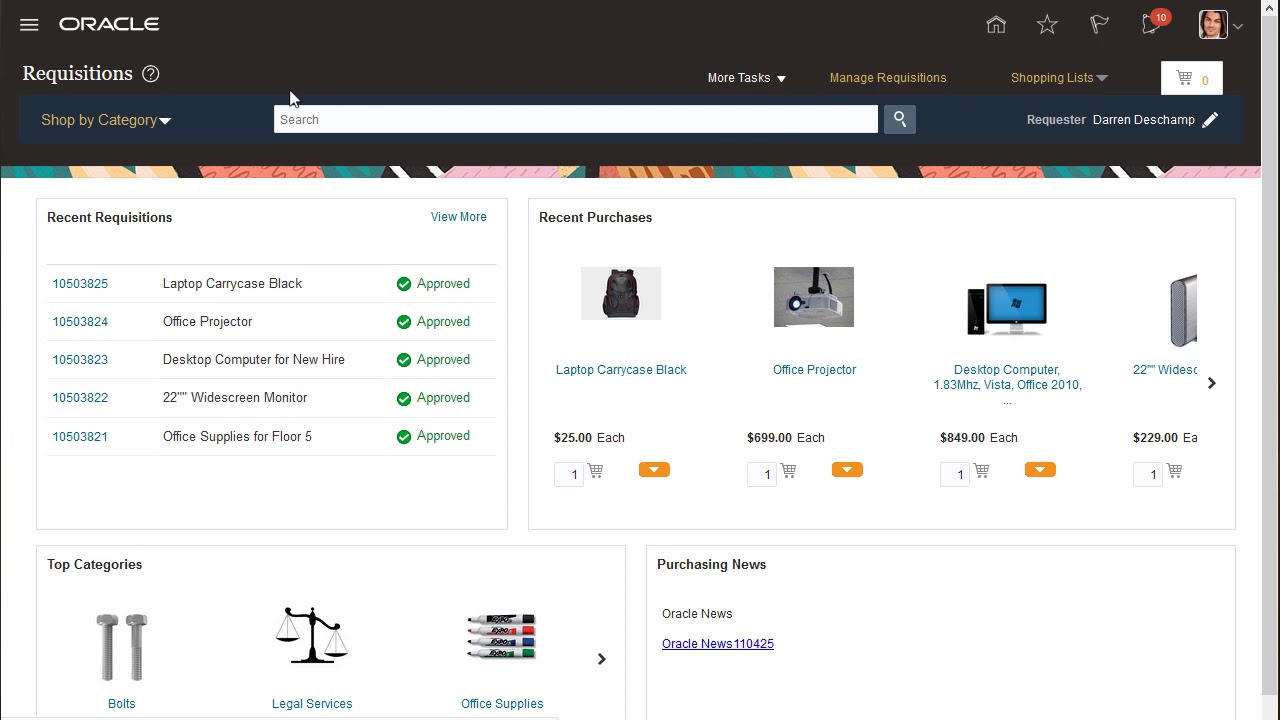Screenshot of the Oracle Webpage:

This detailed image is a screenshot from the Oracle website. At the top, there's a black navigation bar stretching across the screen, featuring the iconic stacked three-line menu icon on the top left. Adjacent to the menu icon is the Oracle logo in their distinct, likely copyrighted, font. To the top right of this black bar is a row of utility icons, including a favorite icon, a flag icon, a user profile icon, a home button, and additional icons that are too small to discern. Beneath the Oracle logo, the header reads "Requisitions" with a small question mark information button positioned next to it.

Centered directly under the black bar lies a white search bar with the placeholder text "Search" and a cursor arrow hovering over it. To the right of the search bar is a gray box containing a white magnifying glass icon, presumably the "search" button. Next to this are a shopping cart icon and several other clickable links, although their labels are too tiny to read clearly.

Just below this banner is a very thin, vibrant strip of colors featuring a variety of hues including pink, red, orange, yellow, teal, green, black, and white. This appears to be a partial backdrop graphic or banner, adding a splash of color to the otherwise minimalist layout. 

The main body of the page is predominantly white with a vertical gray scroll bar on the right edge. The visible content is organized into four rectangular sections, two on the top row and two on the bottom.

The top-left section is titled "Recent Requisitions" and lists several items, each displaying a green checkmark and the word "approved." Each entry includes a requisition number in blue on the left, followed by the item name in the center. For instance, the first item is a "Laptop Carry Case Black," followed by an "Office Projector," and more. Each requisition number, although not fully readable, appears to be a long numeric string.

To the right, in the top-right section titled "Recent Purchases," there are thumbnail images for each purchase accompanied by their names and respective prices. The first thumbnail shows the "Laptop Carry Case Black," priced at $25, followed by an "Office Projector," and a "Desktop Computer" priced at $848. Each entry allows for quantity adjustments, defaulted to 1, with a shopping cart icon and an orange drop-down arrow next to the quantity box.

The left box on the bottom row is labeled "Top Categories," likely listing various product categories, though specific details are not visible. The corresponding right box is titled "Purchasing News," potentially containing updates or information about purchasing or procurement within the platform.